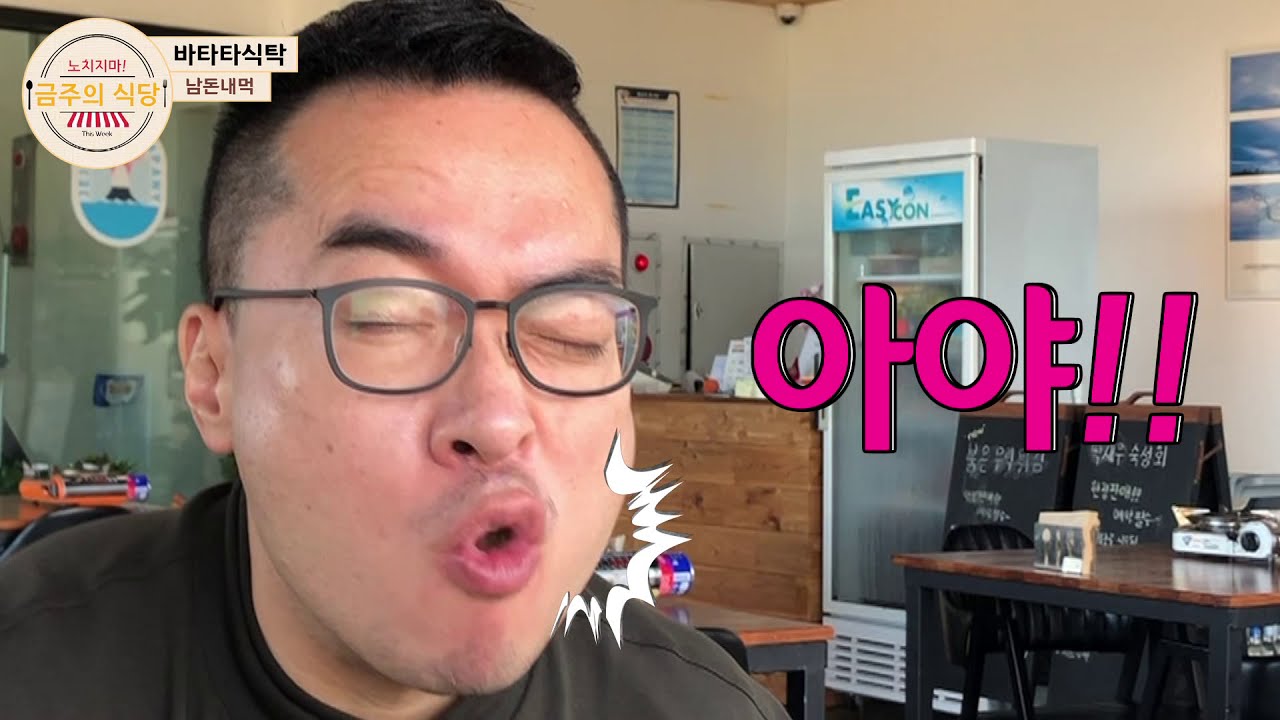The image is a high-quality color photograph of a man with short cropped black hair and a light mustache, wearing black-framed eyeglasses and a green t-shirt. His eyes are closed, and his lips are puckered as if blowing a kiss or whistling. Adding to the playful nature of the photograph, there's an animation of white action marks around his mouth, giving the impression that he is making a 'poof' sound. On the right-hand side of the image is pink text in an unknown foreign language, ending with two exclamation marks. The top left corner features a brand logo with white, yellow, red, and black text, also in an unfamiliar language.

The setting appears to be a well-lit room resembling a cafe or break room. The walls are off-white, transitioning to a yellow hue, and there's a noticeable security camera in the corner where the walls meet. In the background, there is a glass-fronted beverage cooler labeled "LASIKON," partially obscured by a wooden counter space. To the right of the man stands a table with a black base and wooden top. Sandwich boards and various posters or menu boards adorn the walls, adding to the casual atmosphere. A partially visible picture hangs on the wall to the left of the table.